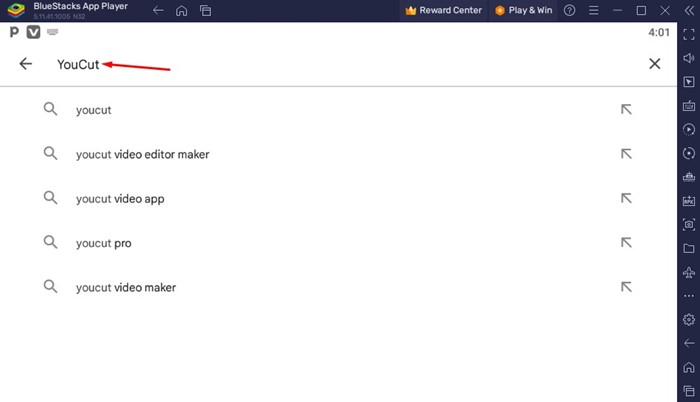The image displays the BlueStacks App Player interface, which prominently features a frame around the main window, particularly along the top and the right side of the screen. At the top left, there are several navigation buttons, including a home button and a link to the reward center labeled "Play and Win." On the right side of this top pane, there are additional buttons and links, such as settings and possibly another home button.

The main section of the screen is dominated by a search engine interface with a white background and black text. The search term "YouCut" (written as a single word with a capital "Y" and "C") has been entered into the search bar. Below the search bar, several search results are displayed, including "YouCut Video Editor Maker," "YouCut Video App," "YouCut Pro," and "YouCut Video Maker." This gives the impression that "YouCut" is related to video editing applications. Despite the somewhat generic appearance of the search engine results page, it is effectively integrated within the BlueStacks App Player interface.